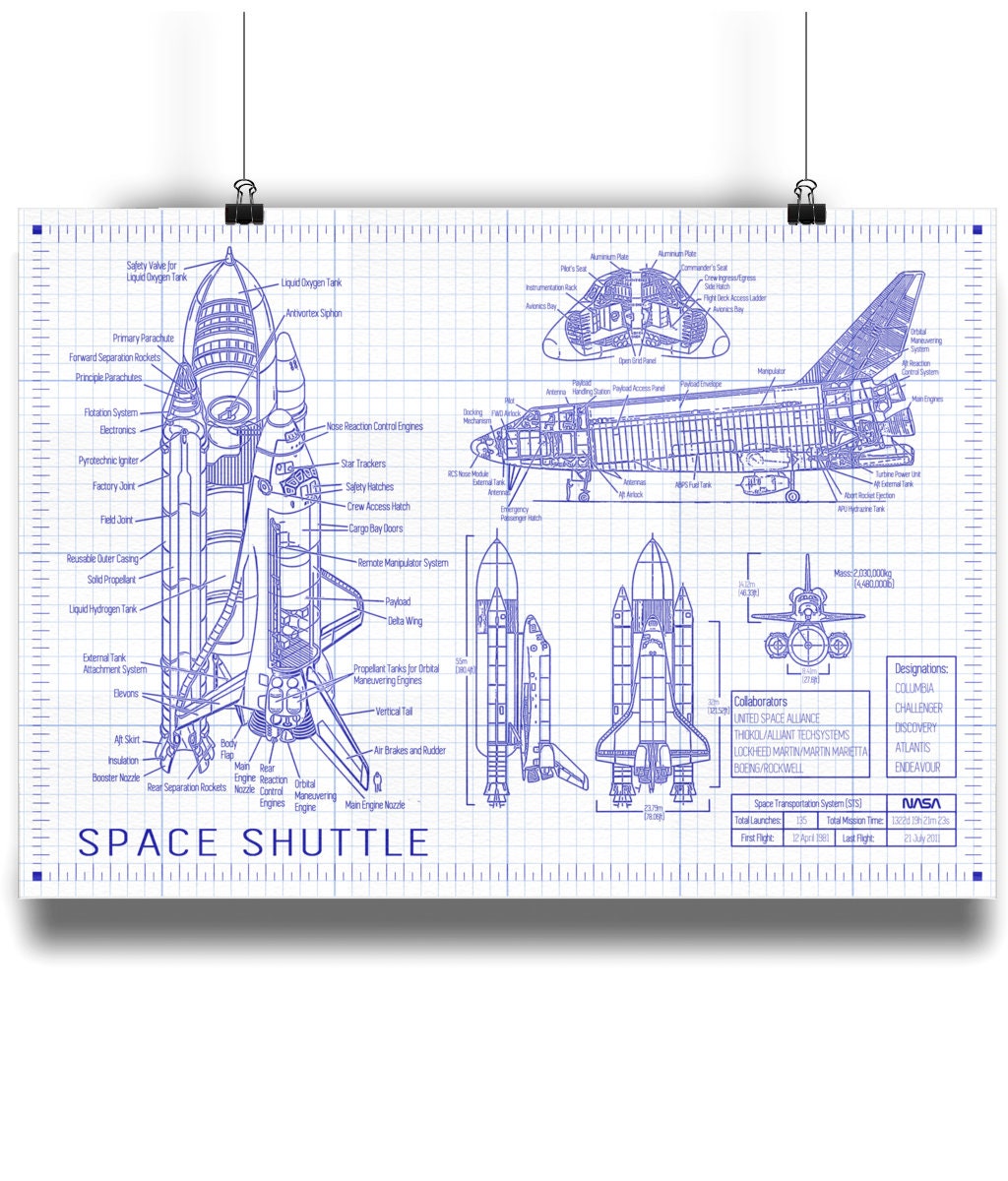The image is a detailed schematic blueprint of the Space Shuttle, meticulously rendered in blue ink on grid paper. A prominent "Space Shuttle" title is clearly visible in the bottom left corner. The primary diagram, occupying the left side, presents a comprehensive, labeled depiction of the Space Shuttle facing upward, detailing its various components from multiple angles. The right side features additional diagrams: the top one illustrates the Shuttle with landing gear extended and positioned vertically, while the two lower diagrams provide alternative views of the Shuttle facing upward. Notably, the image includes textual annotations like "NASA" and possibly "last flight, 21 July 2011", along with designations and collaborator information, though some text remains partially obscured. The illustrations are enhanced with blue arrows and labels identifying key parts of the Shuttle.